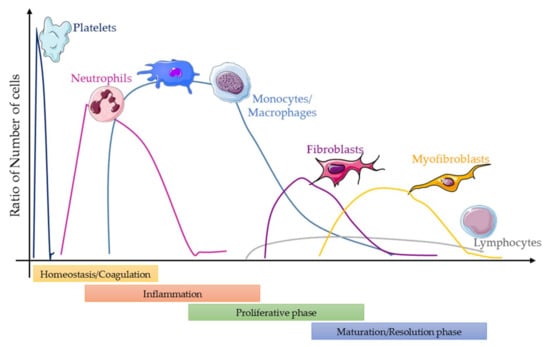The image is a detailed diagram illustrating the ratios of different types of cells across four distinct phases of a scientific process, possibly related to wound healing or tissue regeneration. The diagram is structured on an XY graph, with the Y-axis labeled "Ratio of Number of Cells" and the X-axis divided into four colored phases: homeostasis/coagulation (light orange), inflammation (salmon), proliferative phase (green), and maturation/resolution phase (gray).

Each phase is visually represented with distinct colors and contains specific types of cells. In the homeostasis/coagulation phase, the diagram shows platelets at the top and neutrophils next. Moving right to the inflammation phase, there are monocytes and macrophages. The proliferative phase features fibroblasts and myofibroblasts, while the final maturation/resolution phase contains lymphocytes.

Each cell type is illustrated with unique shapes and colors: platelets, neutrophils with pinkish blobs, monocytes and macrophages with gray and brownish blobs, fibroblasts and myofibroblasts characterized by different shades and shapes, and lymphocytes depicted as blue circles with central grayish-pink blobs. This detailed representation aids in identifying the specific roles and prevalence of each cell type within their respective phases.